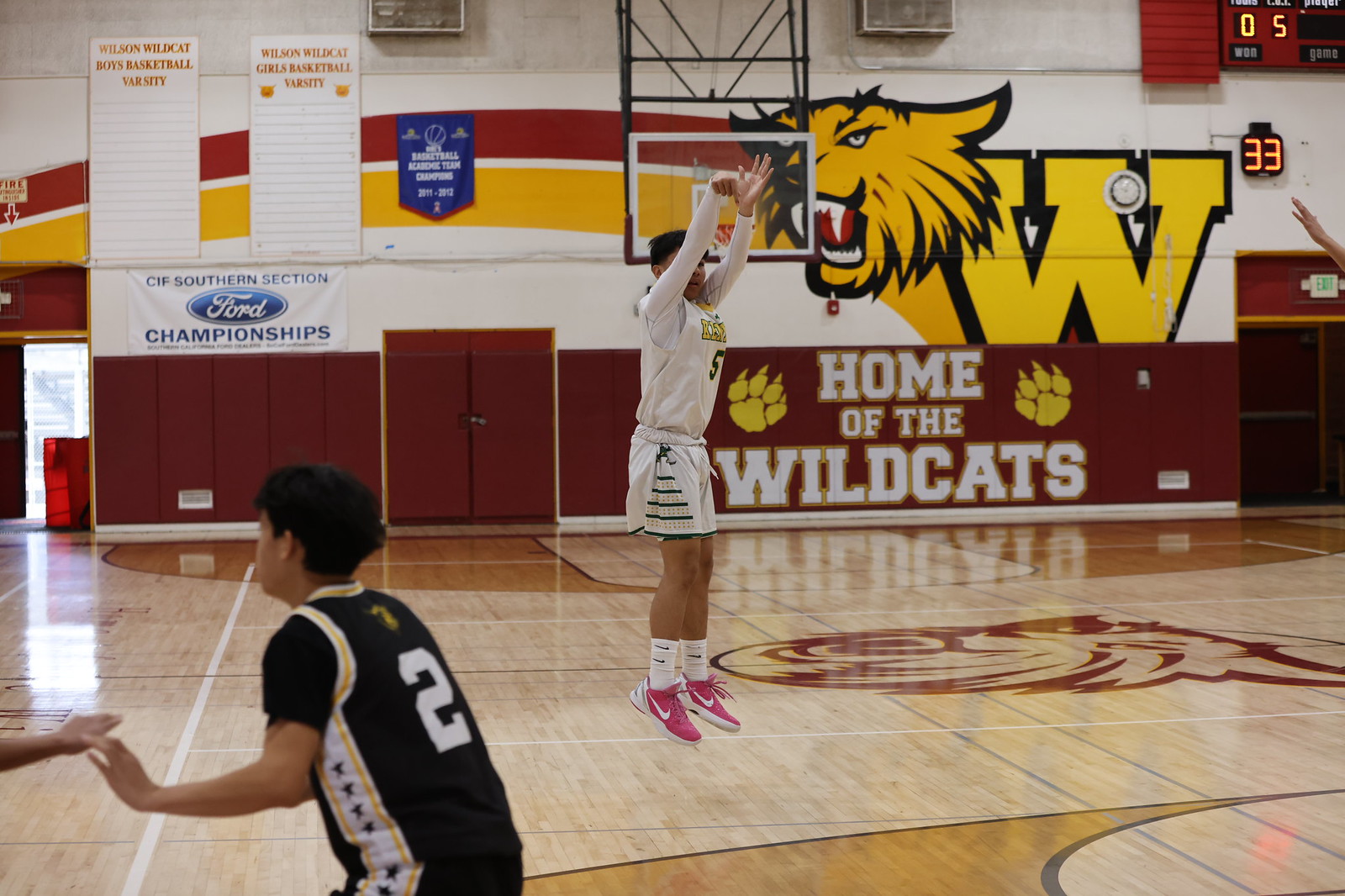In the image set inside a high school gym, two basketball players are captured in the middle of an intense game. Dominating the scene, one player in a white jersey with the number 5, matching long-sleeve shirt, white shorts, white-red Nike shoes, and pink Nikes, is caught mid-jump, with both feet off the ground and arms extended forward, likely having just released a basketball. This player sports a distinctive 90s-style flattop haircut. The opposing player, in a black jersey numbered 2, with a dark complexion and crouched in an athletic stance, is positioned on the lower left side of the court. 

In the background, the gym wall prominently features the logo of a lion with a yellow "W" beneath it, inscribed with "Home of the Wildcats.” To the right section of the wall hangs a scoreboard showing scores of 0 and 5, along with a possible shot clock reading of 33. The wall itself is colored predominantly in white, yellow, and red hues. Further detailed on the left side, there's an indication of the Wilson-Wilcox Girls Basketball Varsity team, noted for its CIF Southern Selection for Championships. Adding to the depth of the scene, an open door appears off to the left side, hinting at a view to the outside, next to a red garbage can.